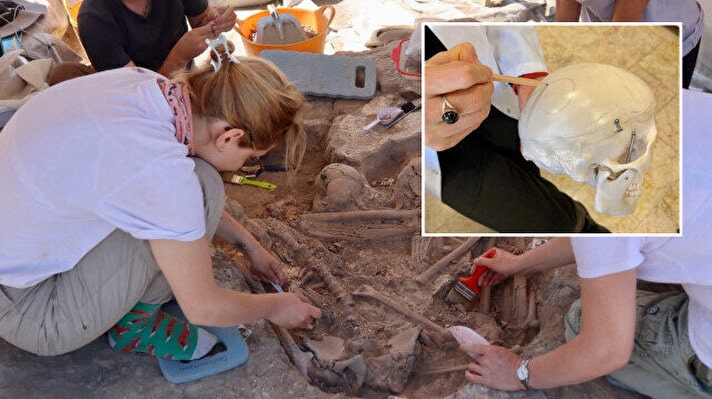The photograph captures an active archaeological dig site with a group of archaeologists meticulously excavating what appear to be human fossils buried in the dirt. Central to the scene is a woman with red hair, wearing a white t-shirt, khaki pants, and bright green socks, carefully examining bones in the ground. Adjacent to her is a man wearing a white shirt, with distinguishable accessories including a watch on his left wrist and a red paintbrush in his right hand, indicating his participation in the excavation. The site is bustling with activity as other archaeologists equipped with various tools—brushes, buckets, and boards—work collaboratively to uncover the fossils.

In the upper right corner of the image, there is an inset photograph bordered in white. This smaller image features a scientist, clad in a lab coat and black pants, holding a polished human skull. The scientist is highlighting a specific area of the skull, which may correspond to the remains being unearthed at the dig site. This thoughtful composition suggests a connection between the in-situ excavation and the analytical processes that follow, providing a deeper context to the archaeological adventure.